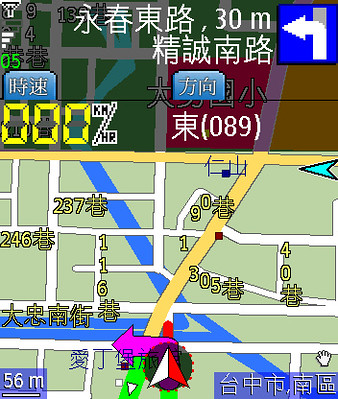The image appears to be a screenshot from a GPS navigation system, featuring a map with detailed graphics reminiscent of a video game interface. The map, rendered in multiple colors, includes a green section at the top and a mix of brown and red on the right. Streets are represented by blue and white lines against a yellow and green background. Overlaying the map, a large white navigation arrow points to the left, while a pink or purple arrow also indicates a left turn. Additionally, there is a red and white arrow pointing upwards. Several labels and numbers are present in an Asian language, possibly Japanese, including a prominent "56M" on the left side. At the top, the display shows a speedometer reading "0, 0, 0 kilometers per hour" with "(089)" beneath it. A small white hand icon is positioned on the right side of the screen, and a teal arrow points left towards the center of the image.